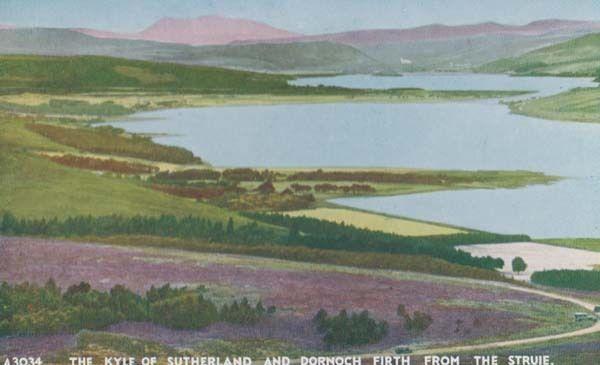This is an image of a painting depicting a serene countryscape viewed from an elevated vantage point. In the foreground, lines of flowers grace the edge of a tranquil lake, their colors muted yet discernable in shades of pink, green, and purple. Surrounding the lake, the lush greenery transitions into a terrain of pink-tinted grasses and plants. The midground is dominated by a large, blue-colored river flanked by verdant banks. In the background, a range of brown hills and mountains rise up against a soft blue sky. Across the bottom of the painting, white text reads: "A3034, the Kyle of Sutherland and Dornoch Firth from the Struie." The overall palette consists of forest green, purple, blue, brown, pink, and beige, creating a harmonious and tranquil scene. This setting, possibly European, showcases the natural beauty of the depicted region.